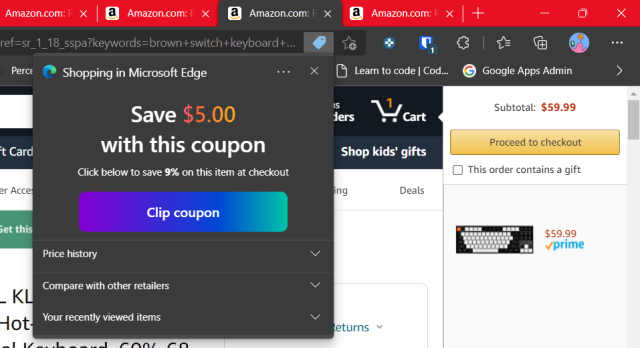![Screenshot from a website showing browser tabs and a shopping interface]

**Top Section:**
- The top of the browser window features a thick red bar about an inch in height, simulating multiple open tabs, similar to those on a computer browser.
- There are several tabs visible:
  - Two red tabs with "amazon.com" written in white text, each featuring a white 'X' icon on the far right side to close it.
  - One black tab with "Amazon" written in red text. Each tab has the Amazon logo on the left, displaying a white box with a black lowercase 'a' and a yellow smile underneath.
  - Adjacent to the black tab, there is another red tab.
  - Following this, a series of icons are located: a white plus symbol, a minus sign, a white box, and another white 'X'.
  
**Middle Section:**
- Below the thick red bar is a slightly thicker gray bar encompassing the address service bar on the left, where website URLs are entered.
- The right side of this bar includes various icons:
  - A blue price tag
  - A white star
  - A blue circle with a white flower
  - A blue bar with a blue circle at the bottom right corner with the white number "1"
  - A white cookie icon with a bite taken out of it
  - Another white star
  - Two white boxes stacked with a white plus symbol on them
  - A blue circle with an icon resembling the top of a pink starfish
  - Three white dots
- Beneath this bar, and encompassed within a drop-down menu on the left, it says "Shopping in Microsoft Edge." To the right of this text is a white 'X' and another set of three white dots.

**Main Section:**
- Centrally located is a prominent notification area:
  - "Save" is written in white.
  - A multicolored gradient from red to yellow to orange forms a money symbol leading into "5.00".
  - Below this, it reads "With this coupon."
  - Further below, white text states, "Click below to save 9% on this item at checkout."
- Underneath this notification:
  - A gradient bar from purple to blue to green features "Coupon" in white text.
  - Below the bar, options such as "Price History" and "Compare with other retailers" are written in white.

**Sidebar:**
- To the right:
  - A white shopping cart icon with a yellow wand inside, labeled with "Cart" in white.
  - Beneath, the heading "Shop Kids Gifts" (in black text), and "Subtotal" (also in black).
  - A red money symbol followed by "59.99."
  - A yellow bar beneath this reading "Proceed to Checkout" in black.
  - An unchecked white box stating "This order contains a gift," written in black.

**Bottom Section:**
- Showing a picture of a black and white keyboard:
  - To the right, a symbol denoting the price at "59.99" in red with a yellow checkmark and the word "Prime" adjacent in blue text.

This detailed scene provides a snapshot of a web interface viewed on Microsoft Edge, featuring shopping details and a section related to coupon savings.